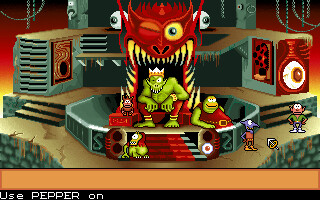This is a small rectangular image of a video game screenshot featuring an older game with pixelated, low-end graphics. The central focus is a large green creature seated on a throne, which is intricately designed to resemble the head of a dragon. The throne is positioned inside the dragon's open mouth, with the seat nestled in the maw. The dragon's head features two large yellow eyes positioned in the background; the right eye is open while the left is closed, both adorned with striking red eyelids. The dragon's mouth reveals long, sharp yellow teeth that add to the fearsome aesthetic.

In the scene, at the bottom left of the stairs leading up to the throne, there is a smaller green creature. On the right side of the image, there is a larger green creature, appearing more prominent than the one at the stairs. Additionally, there are two more creatures positioned to the left, contributing to the menacing atmosphere of the scene. The overall composition evokes a sense of ancient, fantastical conflict, captured with the charm of retro game visuals.